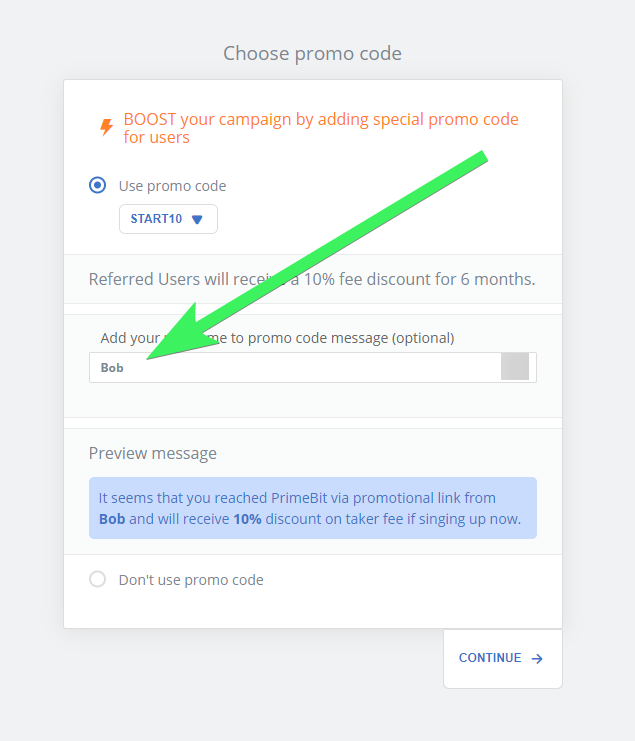This image is a large square screenshot with a gray background. In the center of the screenshot, there is a large white square overlay. At the top of this white square, a message is displayed in red font stating, "Boost your campaign by adding a special promo code for users," accompanied by a lightning bolt icon to the left of the text.

Below this message, to the left, the text “Use promo code” is shown in small blue letters next to a selectable dot. Directly beneath this, a centered drop-down box is set to the value "start10."

Further down, the text “Referred users will receive a 10% fee discount for six months” appears in gray font. Just below, there is a prompt that reads, "Add your message to promo code message (optional)." In the accompanying text box, the word "Bob" has been typed in.

A prominent green arrow is placed diagonally over the image, pointing towards the word "Bob." The arrow's tail is positioned near the top-right corner of the screenshot, while its point targets towards the center-left, emphasizing the word "Bob."

At the bottom of the white square, there's a button labeled "Preview message," under which a blue boxed message reads, "It seems that you have reached PrimeBit via promotional link from Bob and will receive a 10% discount on taker fee if signing up now." This demonstrates the example message that will be shown when "Bob" is entered into the text box.